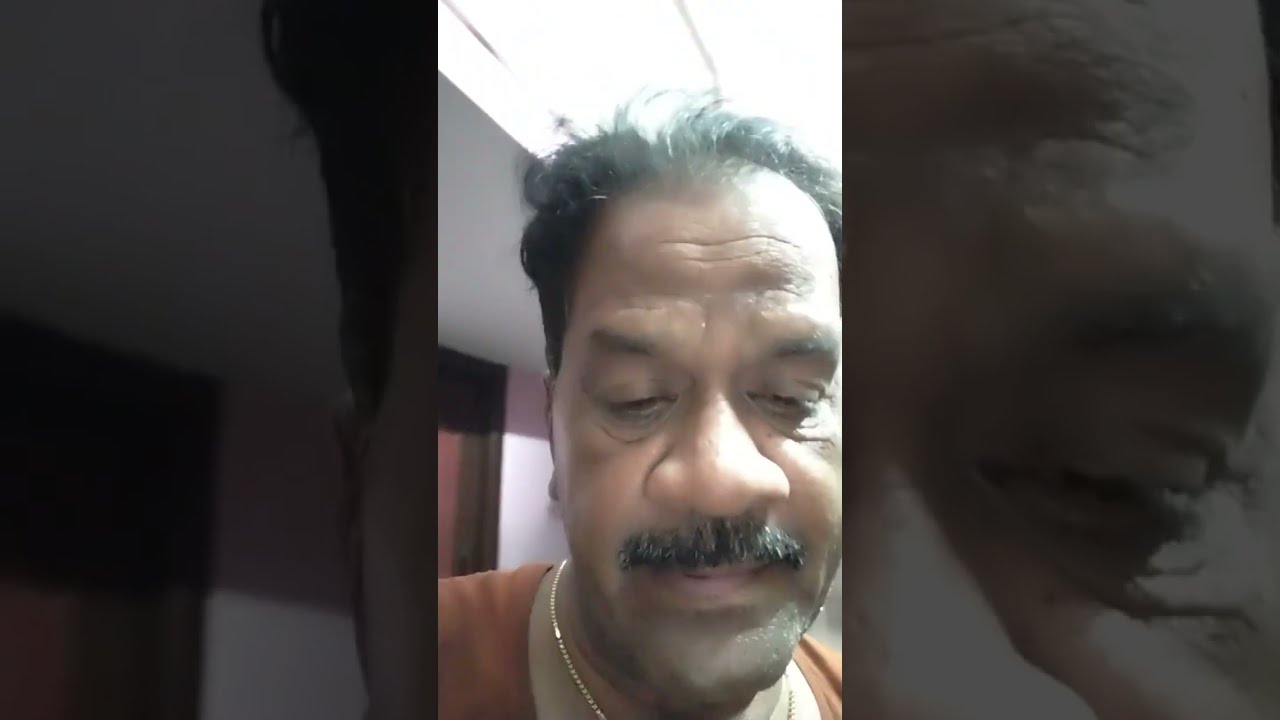A photograph captures an older man, possibly of Indian descent, with a caramel complexion and a predominantly gray mustache mixed with black. His short, slightly disheveled hair is also flecked with gray. The man, centered in the image, wears a thin gold chain around his neck and an orange-red shirt, revealing just his shoulders and neck area. He has a broad nose and appears to be looking down, suggesting he might be reading something. The background is partially visible, predominantly white, with hints of brown and red, including a red doorway in shadow and a bright light source above him, indicating a well-lit room that could resemble an office. The image has a slightly overlapping, darker version of itself on either side, implying it might be a screenshot taken during a video call.